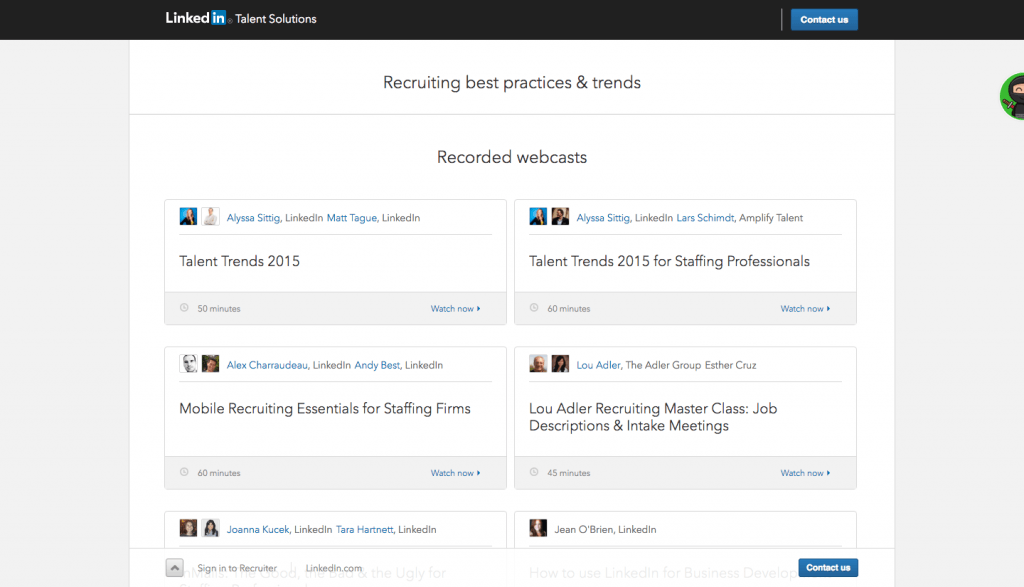This is an image captured from a LinkedIn webpage, specifically from the section titled "LinkedIn Talent Solutions." At the top of the page, there's a black rectangular banner displaying the title in white font. To the right side of this banner, within a blue rectangular button, the phrase "Contact Us" is written in white letters.

Progressing downwards, the background shifts to a gray hue and prominently features a central white rectangle containing detailed information. The first header within this white section reads "Recruiting Best Practices and Trends," followed by a faint gray line that delineates the next portion of the content.

The subsequent section is labeled "Recorded Webcast." This portion includes bullet points that highlight various topics. For instance, under "Talent Trends," there is a mention of "Mobile Recruiting Essentials for Staffing Firms," which is a 60-minute session accessible by clicking "Watch Now." The image also lists contributors Joanna Cusick and Tara Hartnett from LinkedIn, along with an option to "Sign in to Recruiter."

In the upper right-hand corner of this section, there's an emphasis on "Talent Trends 2015 for Staffing Professionals," another 60-minute session available for immediate viewing with a "Watch Now" button. Additionally, Lou Adler from the Adler Group is featured, implying another available video session.

Overall, the image details a well-organized portal for recruiting insights, specifically tailored for staffing professionals seeking the latest trends and practices in the industry.